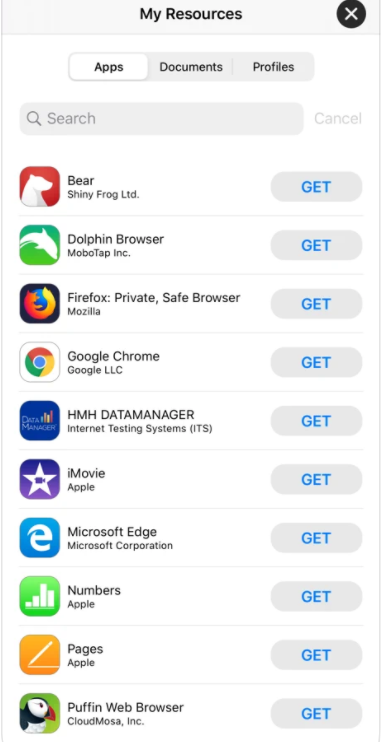The image depicts a vertically-oriented screenshot likely taken on a mobile device, evident from its elongated vertical shape. The top section displays a heading labeled "My Resources" with an 'X' button beside it, suggesting an App Store interface. Below the heading, there are three tabs labeled "Apps," "Documents," and "Profiles," with the "Apps" tab currently selected. Underneath the tabs, a search bar is visible, followed by a list of apps available for installation. Each app entry is accompanied by a gray "GET" button in blue, all-caps font, indicating that the user can download the app by tapping the button. The apps listed sequentially from top to bottom are:

1. Bear
2. Dolphin Browser
3. Firefox Private Safe Browser
4. Google Chrome
5. HMH Data Manager (in all caps)
6. iMovie
7. Microsoft Edge
8. Numbers
9. Pages
10. Puffin Web Browser

In total, there are ten apps displayed on the screen.